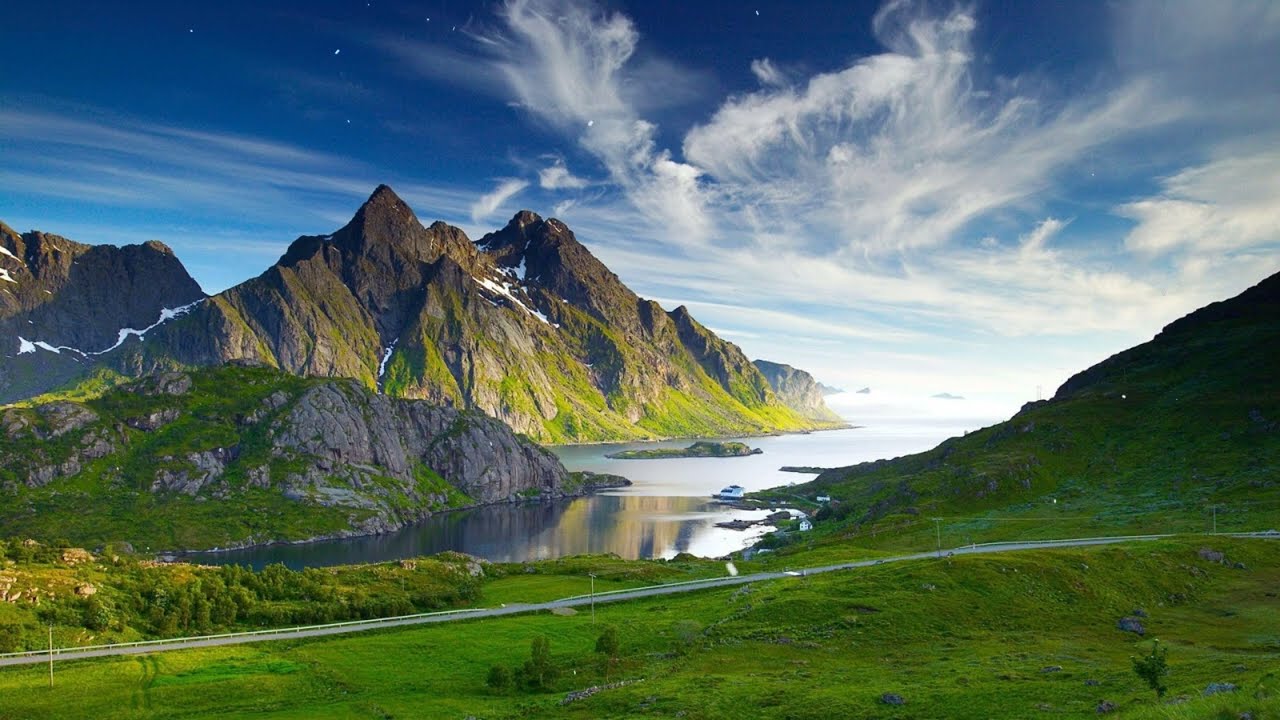A breathtaking, almost surreal landscape photograph captures a stunning mountain range with steep, dark gray peaks contrasting against lush, bright green bases. The scene features a calm inlet in the foreground, formed by rocky hills on either side. A road meanders along the bottom of the image, close to where several cars are parked, and people appear to be fishing at the water's edge. The vivid blue sky above hosts wisps of white clouds scattered throughout and hints of stars becoming visible, suggesting the approaching dusk. Telephone poles run along the road, adding a touch of human presence to the otherwise pristine natural setting. The landscape is further enriched by patches of vibrant green grass on the rocky formations and a serene lake formed by melted snow, capturing the essence of tranquil wilderness.